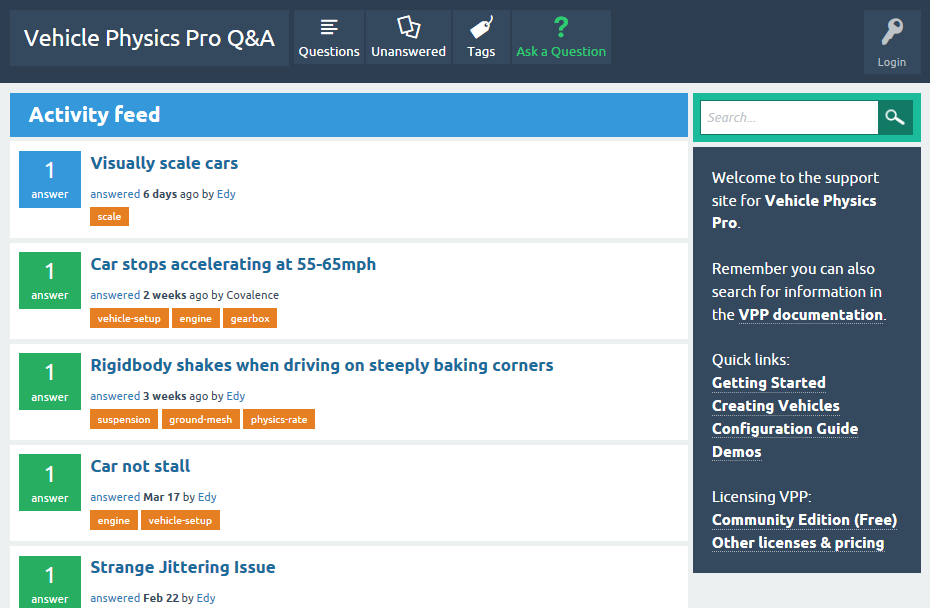This image appears to be an advertisement or informational banner for a support site dedicated to Vehicle Physics Pro. Here’s a detailed description of the layout and elements within the image:

At the very top of the image, there is a horizontal rectangle with a dark blue background. On the left-hand side, within this blue strip, white text reads "Vehicle Physics Pro Q and A," placed inside a lighter blue box outline. Next to this, another lighter blue box displays four single lines in a pattern of long, short, long, short, with the word "Questions" in white underneath. Adjacent to this is a box containing two outlined Polaroid-style photo icons, and below this icon, the text reads "Unanswered." Next to that is a box with a tag icon above the word "Tags" in white. Another box houses a green question mark symbol, and beneath it, the text "Ask a question" appears in green. To the far right, a key icon in light gray is present, labeled "Login" below it.

Beneath this top section, there is a prominent activity feed section occupying most of the left side of the rectangle. Here, a blue background rectangle displays "Activity feed" in white text. Below, a blue square with the number "1" and the word "Answer" is followed by a blue text reading "Visually scale cars." This was answered six days ago by "EDY" (in blue text), with the word "Scale" in an orange rectangle. The feed represents answered questions pertaining to various topics.

Subsequent entries in the activity feed similarly highlight answered questions. For example:
- "Car stops accelerating at 55 to 65 miles per hour," answered two weeks ago by "Covalence," with associated tags in three small orange rectangles: "Vehicle setup," "Engine," and "Gearbox."
- "Rigid body shakes when driving on steeply baking corners," answered three weeks ago by "EDY," tagged as "Suspension," "Ground mesh," and "Physics rate" in orange boxes.
- "Car not stall," answered on March 17th by "EDY," with tags "Engine" and "Vehicle setup."
- "Strange jittering issue," answered on February 22nd by "EDY."

To the right of the activity feed, there is a search bar housed in a green rectangle with a magnifying glass icon.

Adjacent to this, a vertical dark blue rectangle contains a welcome message in white text: "Welcome to the support site for Vehicle Physics Pro." It also invites users to search for information on the "VPP documentation." Below this, the section "Quick links" lists:
- Getting started
- Creating vehicles
- Configuration guide
- Demos

Each link is underlined with a dotted line. Additionally, the text mentions "Licensing VPP" with sub-options: "Community Edition (free)" and "Other licenses and pricing."

This detailed caption outlines the various sections, text, and icons that appear in the image, providing a comprehensive description of the layout and content.